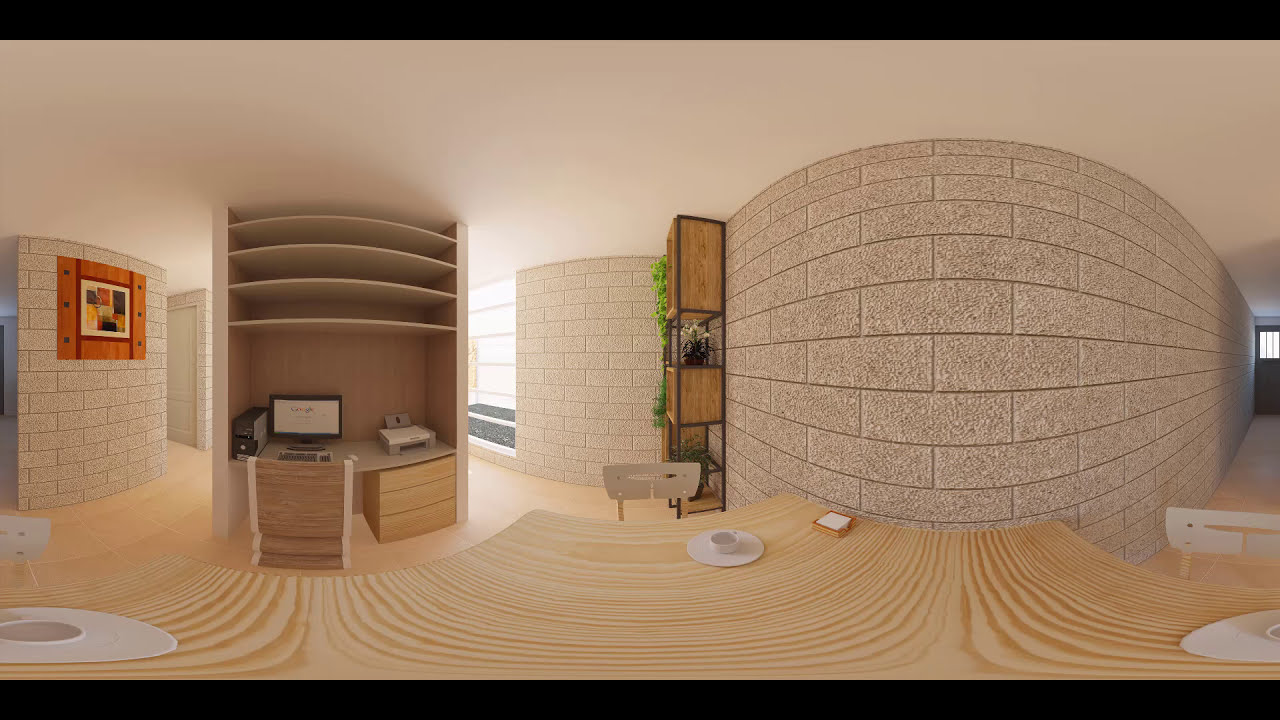This detailed image captures the interior of a living area, potentially a 3D-rendered scene with noticeable fish-eye distortion, lending a curvy, somewhat surreal appearance. The room features distinct light gray, brick-style walls, segmented into horizontal rectangles with visible grout lines. 

The focal point is a well-organized desk area on the left, illuminated by light streaming through a window behind it. The desk, topped with a tan surface, holds a computer monitor, desktop computer, printer, and keyboard. Above are several rows of built-in shelves. Adjacent to the desk is a light brown or tan chair, neatly tucked in. 

On the left wall hangs an eye-catching abstract painting with an orange frame. The light wood grain-patterned carpet overlays a seemingly new, fresh hardwood floor, adding warmth to the space. 

In the middle of the room, there's a table, perhaps with a plywood finish, topped with a white mug on a saucer. Notably, the floor pattern is curvy with multiple lines, enhancing the room's distorted aesthetic. The overall color palette leans toward light browns, tans, and grays, contributing to a cohesive and modern look.